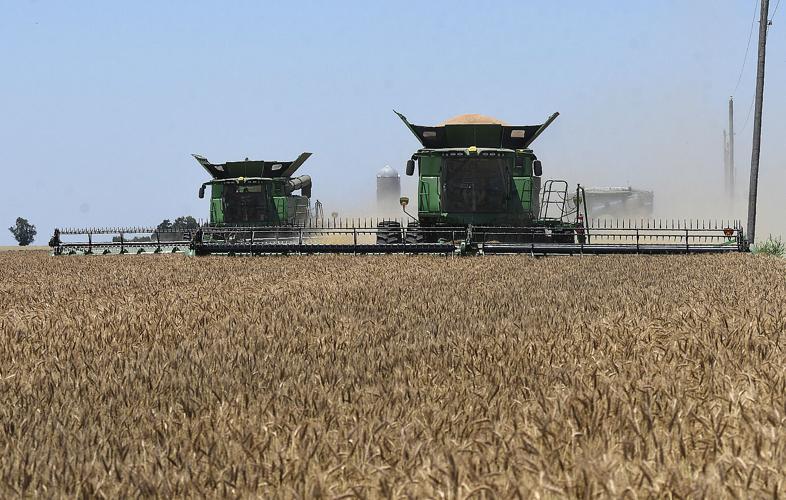In this vibrant outdoor scene, three large green combines are actively harvesting a field of golden wheat under a perfectly blue sky. The combines, with their black front attachments, are efficiently mowing the wheat and collecting it. One of the combines on the right is emptying a full load of wheat into a nearby trailer, with golden grains spilling over the top. Another combine on the left mirrors the design but is still at work without a trailer. In the background, a tall grain bin with a white dome lid stands prominently, beside a line of utility poles on the right and a cluster of trees on the left. The scene captures the essence of the harvest, with the combines kicking up dust as they move through the amber waves of grain.